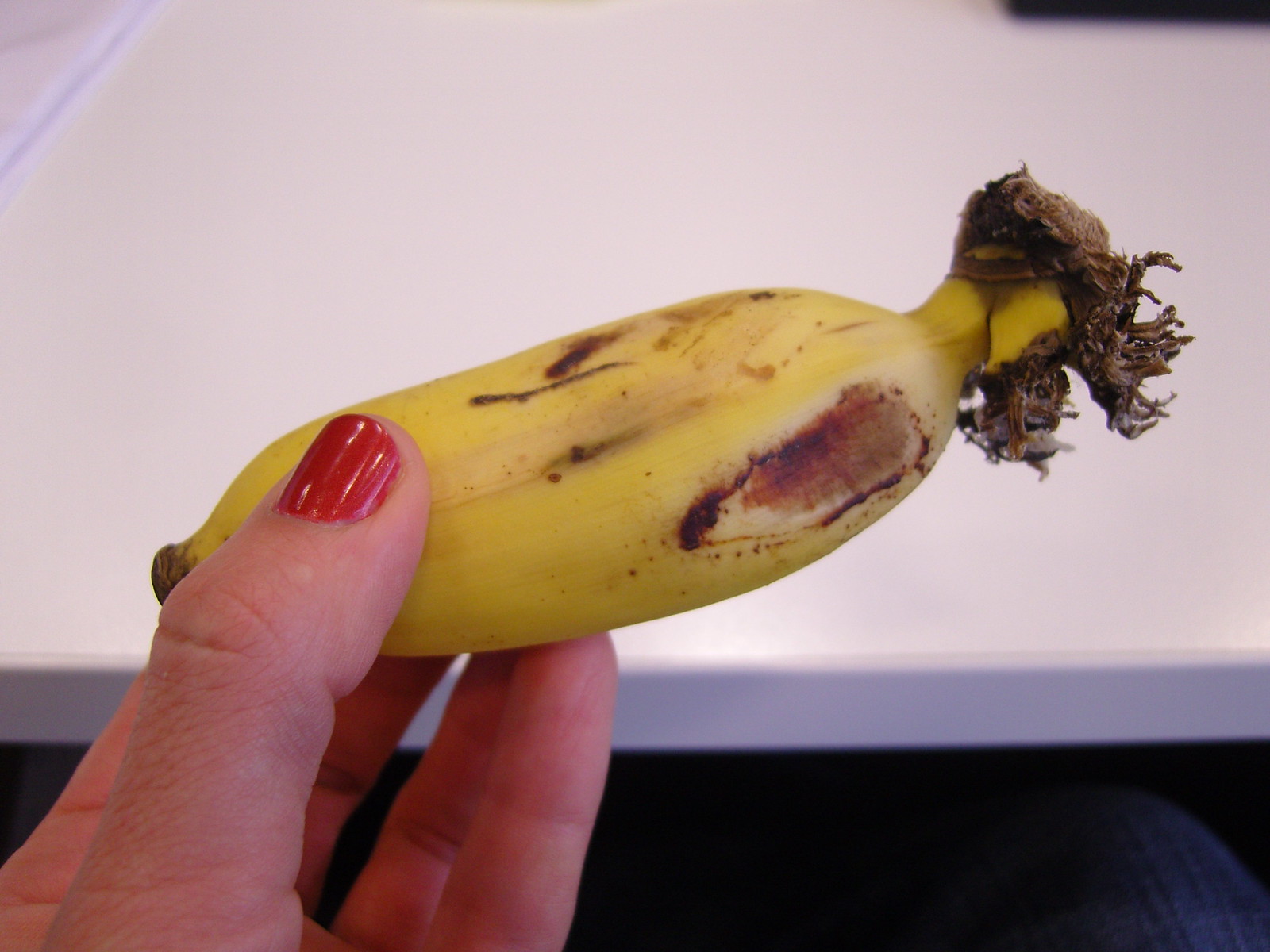In the center of the image, a hand is holding a very short banana. The photograph is predominantly filled with a white table or countertop occupying the top three-quarters of the image. The bottom quarter features a dark background, which appears to be the floor visible beneath the edge of the table. From the bottom left side of the frame, fingers of a left hand emerge, visible from the bottom joint of the fingers to the tips. The pinky, ring, and middle fingers cradle the banana, positioning it diagonally across the image from left to right, with the thumbnail (painted in red nail polish) facing up. The banana, roughly three to four inches in length, has a notably bushy stem and a small bruise on the right side, which bears a reddish hue. This blemish makes it difficult to determine whether the banana itself has a convex area or if it's merely a mark on the skin. No other parts of the person holding the banana are visible in the image.